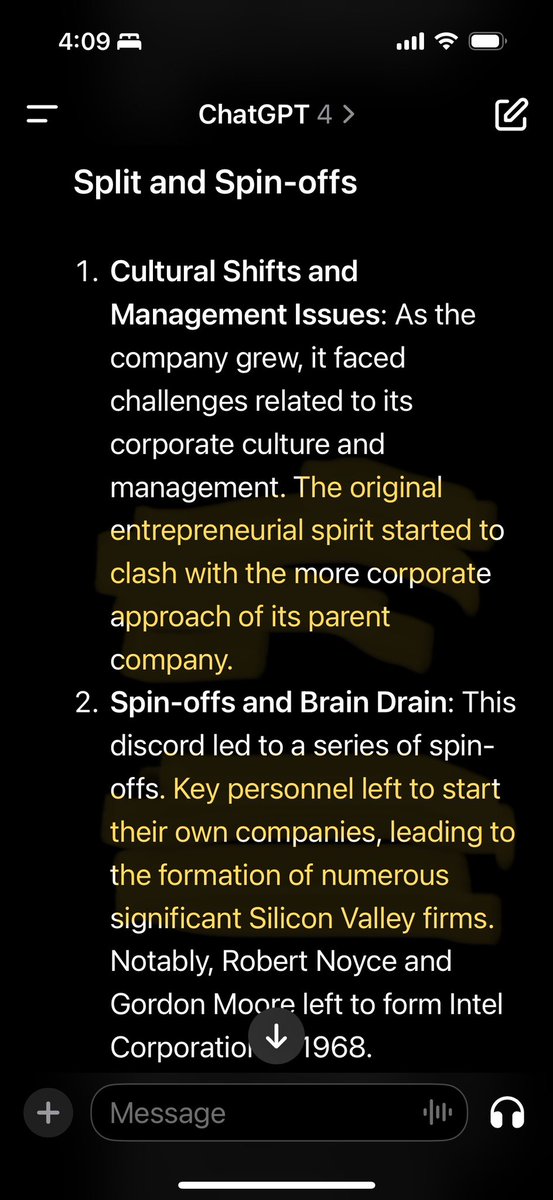This image is a detailed screenshot of a smartphone displaying a Chat GPT-4 conversation with a black background and white text discussing "split and spinoffs." At the top left, the time is 4:09, indicating bedtime mode with a bed symbol. The top right shows icons for a tornado (representing Wi-Fi), a battery, and a cell tower signal. The text is divided into two sections: "1. Cultural shifts and management issues," describing how the original entrepreneurial spirit clashed with the corporate culture of the parent company (highlighted in yellow), and "2. Spinoffs and brain drain," explaining how key personnel left to form significant companies like Intel Corporation in 1968 (highlighted in yellow). The interface also features a message bubble, a headphone symbol on the right, and a plus sign on the left.